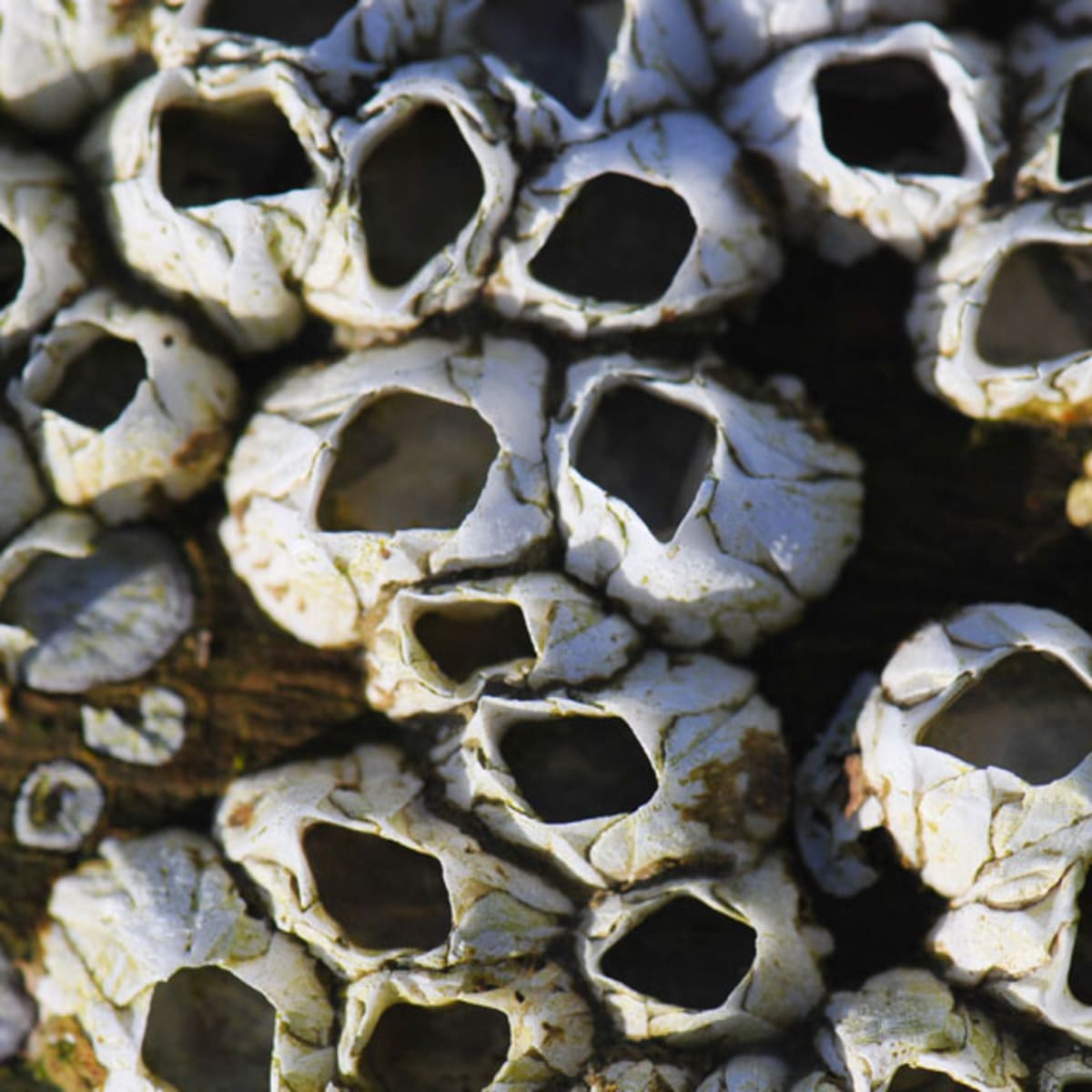This high-resolution, extreme close-up photo captures a fascinating scene of what appear to be barnacles or hollowed-out rock formations against a dark brown sandy background. The objects are white and circular, with various sizes and irregular shapes—some resembling imperfect ovals or thin, wide forms. Each object has an open top revealing a dark, black interior, with some openings being circular, oval, or even square. The white surfaces are marbleized with green mossy sections and veins, and exhibit weathered cracks and splotches of brown. Sunlight highlights their bleached, eggshell-like texture, suggesting they’ve been exposed to the elements for some time. The entire composition, viewed from above, creates an intriguing contrast between the pristine white formations and the dark sand, capturing the natural beauty and complexity of these unique structures.